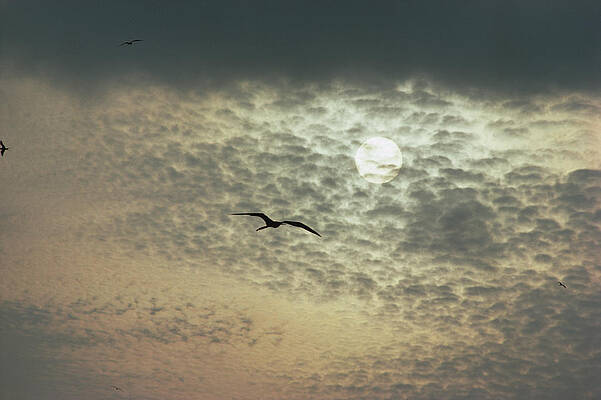The image depicts a captivating scene where a black silhouetted bird soars gracefully in the sky, its wings fully extended. The photograph is taken from the ground looking up, featuring a sky layered with various shades of grey and dark clouds. Dominating the center of the image is a luminous full celestial body, possibly the sun or the moon, partially obscured by wispy clouds. The top half of the sky transitions from a deep grey to near-black, while the lower part bathed in a soft peach light gradually fades into darker grey tones. The atmospheric lighting suggests that it's either dusk or near sunset. The contrast between the stark silhouette of the bird and the gradient sky, enriched by the interplay of light and shadow, adds a dramatic and serene quality to the scene.